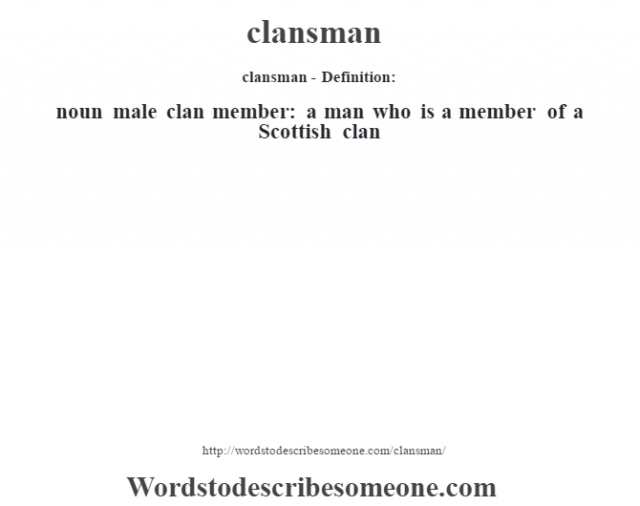The image displays black text on a plain white background, centered across six lines. At the top, it features the word "clansmen" in lowercase. Below it, a smaller line reads "Clansmen definition: noun," with the D in "definition" capitalized. Further down, the text continues in lowercase, defining "clansmen" as "male clan member: a man who is a member of a Scottish clan," with the S in "Scottish" capitalized. The bottom of the image shows two URLs in black text. The first, in very small print, reads "http://words2describesomeone.com/clansmen." Directly below, a larger version of the URL, "words2describesomeone.com," is displayed. The overall layout is minimalist, with substantial white space between the definition and the URLs.